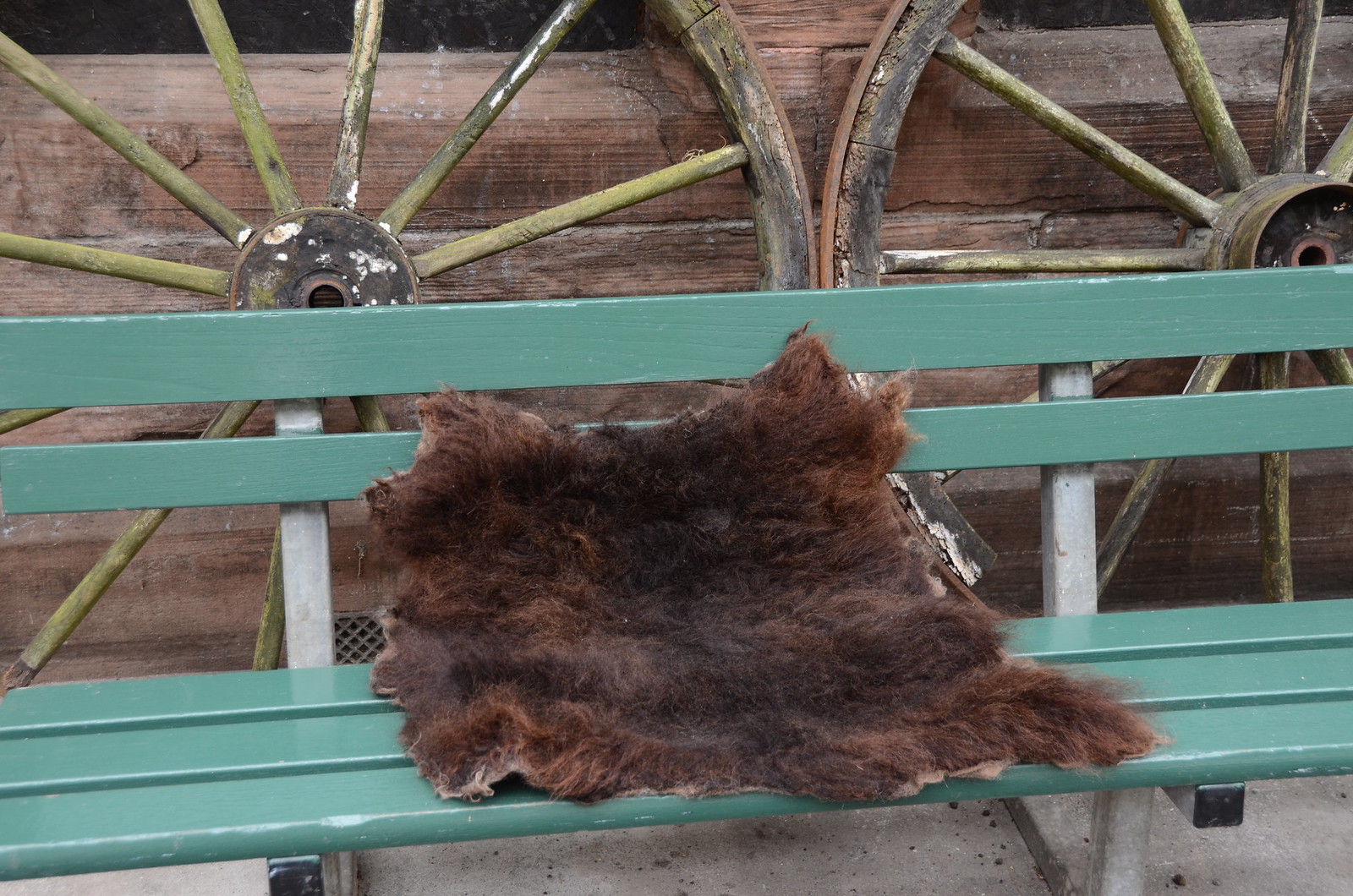The photograph captures a scene centered on a long, green wooden park bench with metal stanchions, partially cut off at the ends. Draped across the middle of the bench is a dark brown animal pelt, possibly a fox skin, which appears shriveled and brittle around the edges. This suggests the tanning process may not have been successful, leaving the fur fragile. Directly behind the bench are two large wagon wheels with wooden spokes and rims encased in metal. The wheels seem to be part of an old cart. Encircling this scene is a rough wooden fence or wall made of horizontally-placed boards. The flooring beneath the bench and structures is gray concrete, adding to the rustic outdoor setting—likely captured in the middle of the day given the lighting. The overall image is marked by an assortment of natural colors: green, brown, black, and gray, contributing to the earthy, historical ambiance.